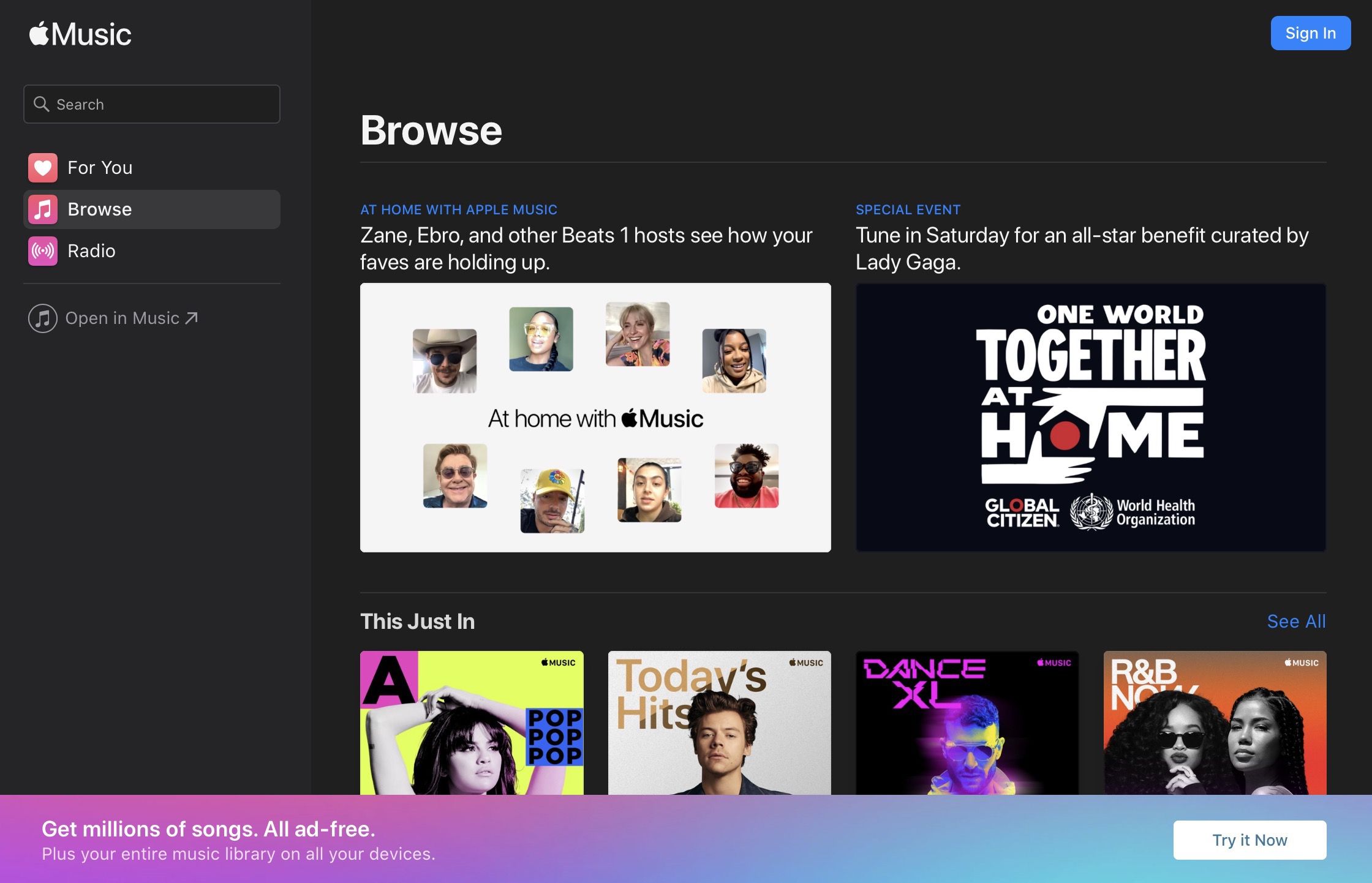This digital image showcases the interface of Apple Music, highlighting its diverse features and offerings. Prominently displayed are pictures of musical artists and album covers, providing a vibrant mosaic of the platform’s content. Key navigational tabs such as the "For You" tab, "Browse" option, and "Radio" option are clearly visible, illustrating easy access to personalized music and curated content. 

The image features a section titled "At Home with Apple Music," showcasing artists like Zayn and Ebro alongside other Beats-related content, inviting users to see how their favorite musicians are engaging with fans. Several images of different people add a dynamic feel to this segment.

A notable highlight is the advertisement for a special event: "Tune In Saturday for an all-star benefit curated by Lady Gaga," promoting the "One World: Together at Home" event, jointly organized by Global Citizen and the World Health Organization. 

In the upper right corner, there's a blue and white "Sign In" button, ensuring easy access for users to log into their accounts. The caption also promotes the service's perks, stating, "Get millions of songs all ad-free, plus your entire music library, all on your devices," emphasizing the platform's extensive, ad-free music library.

Another call-to-action, "Try It Now," encourages new users to explore Apple Music. Featured prominently is an album cover of Harry Styles under the "Today's Hits" category, inviting listeners to tune into popular contemporary music.